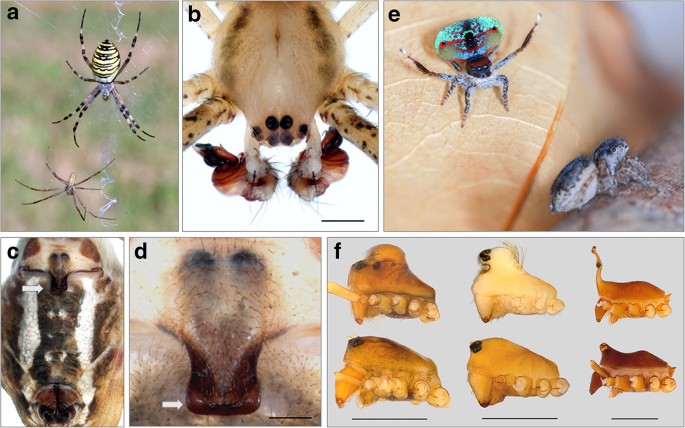The composite image features six labeled frames (A, B, C, D, E, and F), primarily focusing on various close-up photographs of spiders or insects displaying different aspects and angles. 

In frame A, there is a spider on a web with a yellow and black striped insect slightly out of focus behind it. Frame B presents a detailed, zoomed-in view of a brown and black animal, likely a spider. Frame C highlights the intricate face of another spider. Frame D showcases a different perspective of a spider's head. Frame E depicts a pair of spiders as seen through a microscope, possibly on a surface resembling skin. Lastly, frame F shows the mouthpart of a spider or insect, detailing broken teeth and possibly fins. The colors of the spiders range from yellow and black to brown, red, white, and blue, collectively illustrating the diverse anatomy and environments of these arachnids.